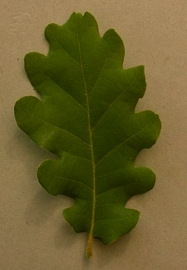The image depicts a single green leaf with rounded edges, characterized by eleven distinct lobes. The leaf, bearing a central vein with several branching veins, lies flat on a smooth, off-white or tan-colored surface, likely a countertop or table. The background has no discernible texture or wood grain, and the leaf, possibly resembling an oak leaf, is elongated and exhibits a sequence of rounded bumps along its sides. This photograph focuses solely on the green leaf against an unobtrusive background, highlighting the intricate details of the leaf’s veining and shape.